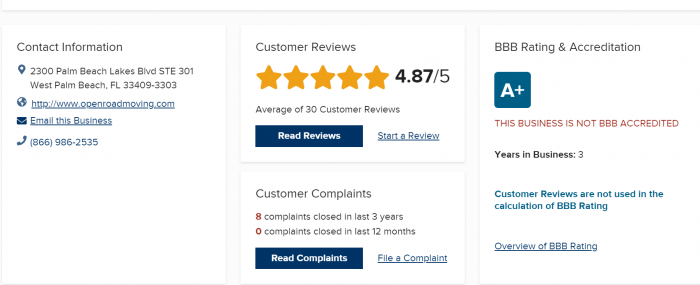Detailed Caption:

The image showcases a well-organized layout divided into three horizontal sections, each providing key information about a business. The first section on the left contains the business's contact information. The business name listed is "Open Road Moving," and it is located in West Palm Beach, Florida. Their website is openroadmoving.com.

The middle section features customer feedback. It highlights an impressive average rating of 4.87 stars out of 5, based on 30 customer reviews, reflecting high customer satisfaction. Located just below this is the customer complaints section, which indicates that the business has resolved eight complaints in the last three years.

The final section on the right focuses on the Better Business Bureau (BBB) ratings and accreditation. The business boasts an A+ rating from the BBB, which signifies excellent business practices. However, it is noted that "Open Road Moving" is not currently BBB accredited despite the high rating.